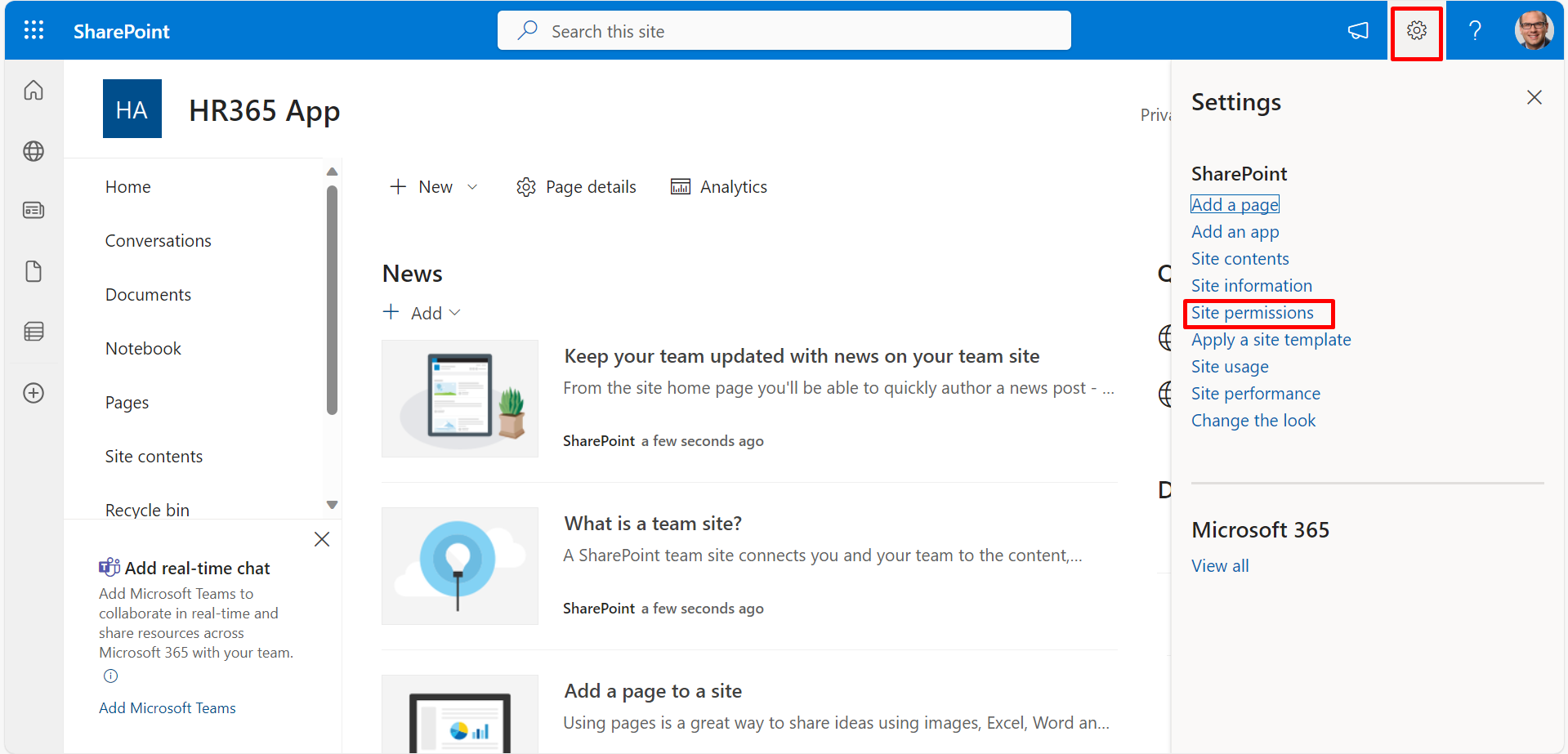The image showcases a SharePoint interface captured from a screen. At the top of the page, the SharePoint logo is clearly visible, immediately followed by a prominent search bar in the middle section. To the right of this central area, there is an icon resembling a megaphone, presumably to amplify your voice or announcements. Adjacent to this, a gear icon, highlighted by a red square, signifies access to settings. Additionally, an area labeled "Site permissions" is also encircled in red, located on the settings page to the right.

In the upper portion of the screen, the title "HR 365 App" is prominently displayed in white print against a navy background, next to the letters "HA". Below this header, navigation links are listed, including Home, Conversations, Documents, Notebook, Pages, Site Contents, and Recycle Bin. Moving further to the right, there is a "News" section accompanied by a "+ Add" button and instructions stating, "Keep your team updated with news on your team site." Additional guidance includes, "What is a team site?" and "Add a page to a site."

On the right-hand side, under the settings section, there are references to SharePoints and an option to "View all" under Microsoft 365, facilitating easier access to further resources.